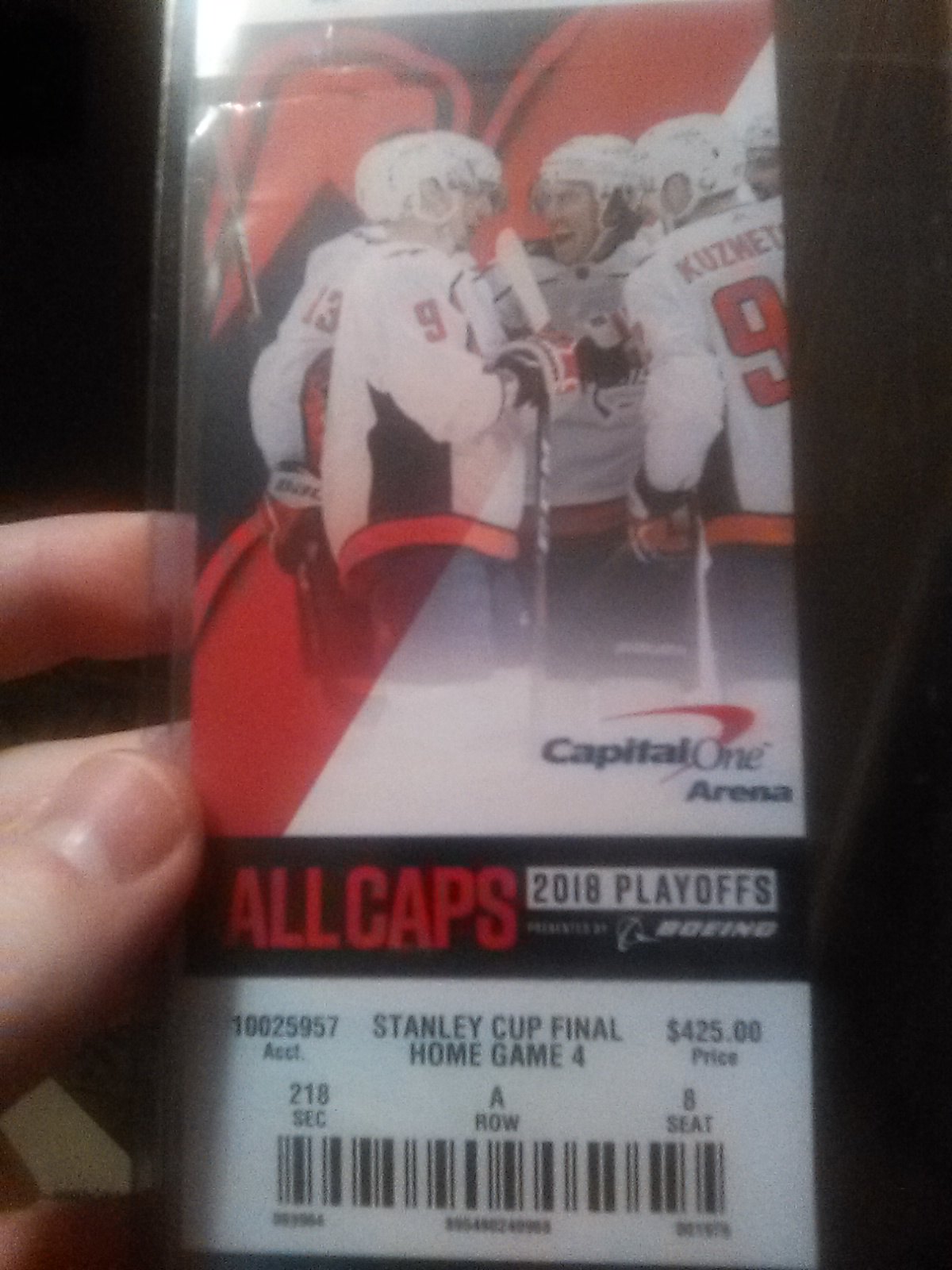The image is a detailed photograph of a ticket for a 2018 Stanley Cup Final game at Capital One Arena. The ticket is being held upright in the left hand of a person, evident by the visibility of their left thumb and index fingers. The ticket itself has a digitally created image at the top depicting a group of hockey players in white, red, and black uniforms with white helmets and black pants, celebrating together. Below this, in red all caps font, is the text "2018 PLAYOFFS," and nearby, the Capital One Arena logo, featuring a red arc, is prominently displayed. Further down, a white box contains the information "Stanley Cup Final Home Game 4," alongside additional demographic and price details, including a barcode and seat information, which specifies Section 210, Row A, Seat 8. The ticket is encased in plastic, suggesting that it is preserved as a keepsake. The colors on the ticket predominantly include black, red, and white, and the background of the photo appears to be an indoor setting.